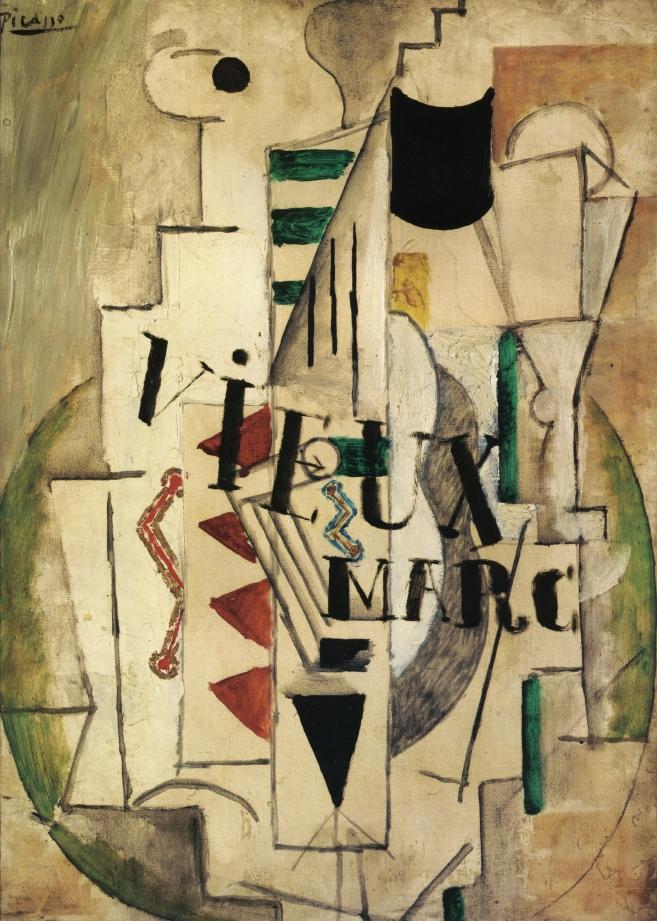This abstract image presents a complex collage of diverse shapes and colors, suggestive of modernist influences, potentially reminiscent of Picasso. Dominating the background, the left side features a blend of beige, brown, and green hues, while the right side is predominantly brown. Central to the composition is a long rectangular shape outlined in grey, enclosing a black inverted triangle. At its top are three black vertical lines, juxtaposed by three green horizontal lines emerging from the top left. Just to the left of this central rectangle are four brown rectangles pointing left. Superimposed on the image are two words in bold black text, "V-I-E-U-X M-A-R-C" or possibly "V-I-E-U-X M-A-R-Z." Throughout the piece, a rich palette including greens, blacks, tans, browns, whites, reds, blues, yellows, and oranges, emerges from the overlapping shapes. Additionally, a signature that reads "Picasso" appears in the top left, suggesting a tribute to the famous artist. The design occupies the entire canvas, with no blank space, making it a striking piece that could easily belong in a museum.